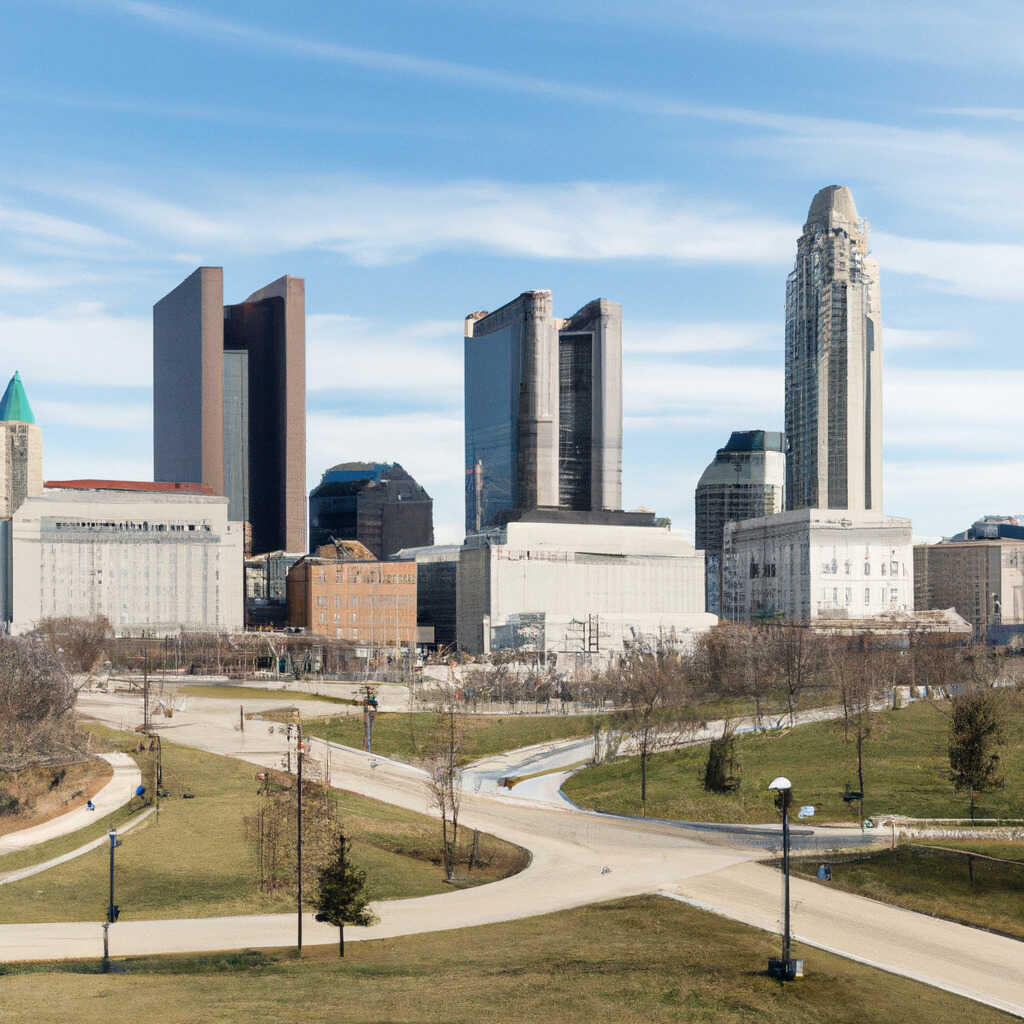This daytime photo captures a downtown cityscape, likely from a mid-sized town a couple of decades ago. The skyline features several high-rises spread out, with the tallest building on the far right boasting a rounded top and stretching into the clear blue sky. Wispy white clouds can be seen above, adding depth to the scene. In contrast to the tall structures, there are older, shorter commercial buildings below, resembling warehouses and ranging from seven to eight stories high. These buildings are mostly square or rectangular and vary in color, including white and an orangish hue. At the base of the photograph, a park area is visible, adorned with walking trails, tall black lampposts, and patches of green grass. The park's trees are mostly thin and scraggly, many appearing withered without leaves, suggesting it might be fall or a time when foliage is sparse. However, one tree in the foreground is fully covered, adding a touch of greenery to the scene. Overall, the image portrays a serene urban environment blending nature and architecture.